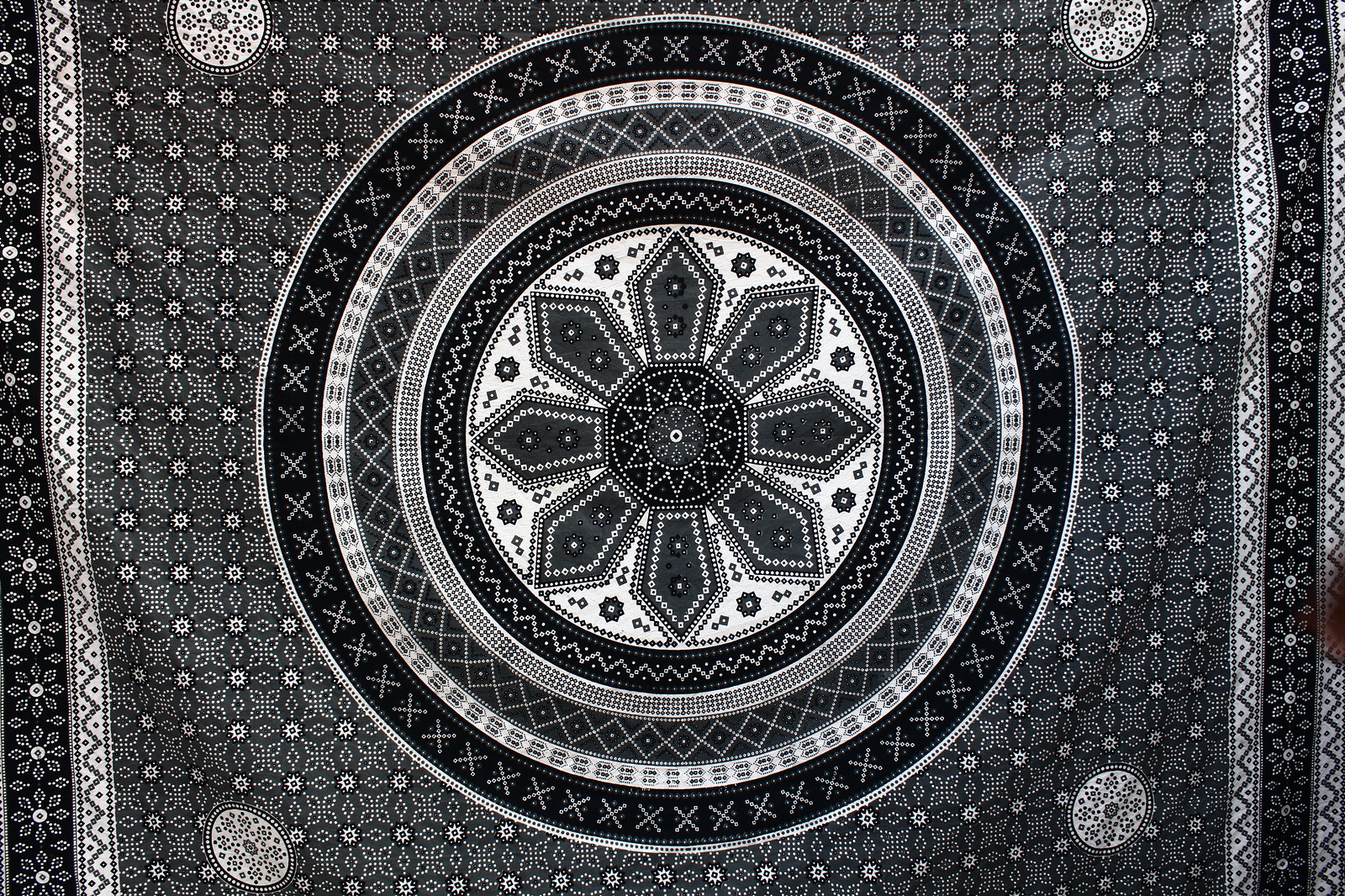This photograph captures an expansive, intricately designed tapestry predominantly in shades of black, gray, and white. Dominating the center is a large, intricately detailed circle featuring an eight-pointed star with an inner circle adorned with spear-like shapes radiating outwards. The subsequent circles around this central motif exhibit a range of patterns: a black and white sunburst, followed by layers of dots, petals that resemble a mandala, and various zigzag and brick-like patterns. The tapestry is further accentuated by additional concentric circles with designs such as black mandalas, diamond-shaped zigzags with central white circles, and large segments of dark gray bordered by white X’s. The entire piece rests on a background of dark gray with white mandala flowers and lighter gray accents. In each corner (top right, bottom right, top left, and bottom left) is a white circle filled with black dots. Framing the tapestry are borders of white with gray zigzags and black with white floral patterns, adding to the overall complexity and visual richness of the piece.